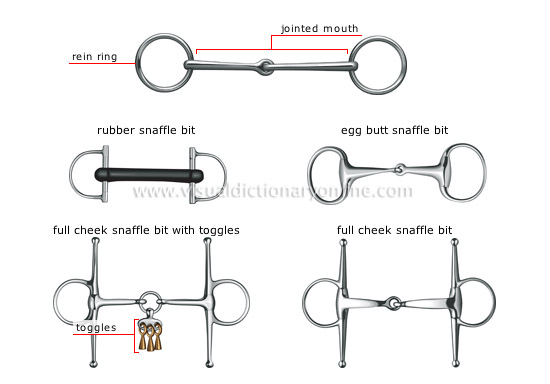The image showcases five distinct types of metal horse bits against a white background, with all the metal predominantly gray. Centered around the watermark "www.visualdictionaryonline.com," the image is labeled with detailed descriptions. At the top, a bit labeled as "jointed mouth" has a "rain ring" on the left side, connected to another ring by a central metal piece. Red lines point to this central area. Beneath this, the "rubber snaffle bit," distinguishable by a black rubber component connecting two metal pieces, is identified. To the right, an "egg butt snaffle bit" is described. On the bottom left, a "full cheek snaffle bit with toggles" features three brass-colored toggles, each labeled with red lines. Finally, the "full cheek snaffle bit" appears again in the bottom right corner. The image utilizes a color scheme of black, white, red, silver, and copper, and the objects are meticulously arranged but not centered, giving a detailed and instructional presentation.